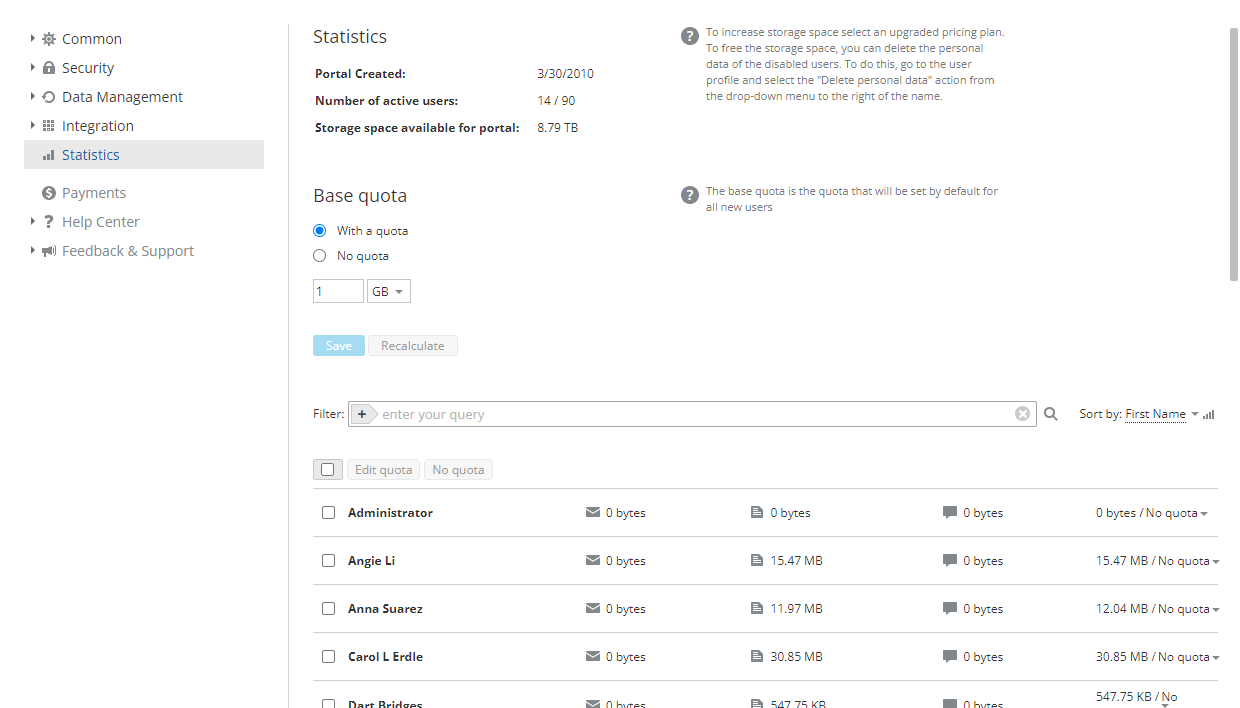The image depicts a comprehensive data management interface with multiple functionalities and sections. On the left side, there's a navigation menu featuring an arrow pointing at "Common Security Data Management Integration." Below this section, the menu lists "Statistics," "Payments," "Help Center," and "Feedback and Support," each accompanied by relevant icons—a lock for security, bar charts for statistics, a dollar sign for payments, a question mark for the Help Center, and a speech bubble for feedback and support.

At the center of the interface, the "Statistics" panel is prominently displayed. It shows that a portal was created on a specific date (not clearly readable), listing 14 active users out of a possible 90. The available storage space for the portal is indicated as 8.79 TB (terabytes). Beneath this, there's a setting for storage quotas, with options for "With a quota" and "No quota," where "With a quota" is selected, marked by a filled blue circle.

Further down, two input boxes allow users to specify data amounts, with one box filled with the number "1" and the other specifying the unit "GB" (gigabytes). There are two buttons adjacent to these input fields: a blue "Save" button and a "Calculate" button.

A filter bar, equipped with a search function and a magnifying glass icon, allows users to look up specific information. Below the filter bar, a list of administrators is displayed—ANGU, Anna Suarez, and Carol L. Erdl—all showing "zero bytes" of data moved next to their names, along with additional details of their data usage next to each name.

To the right of the statistics panel, there's a paragraph of text with a question mark icon next to it, potentially representing a help tooltip or further information. Below this, another line of text with a question mark icon is present, although it's too small to read clearly.